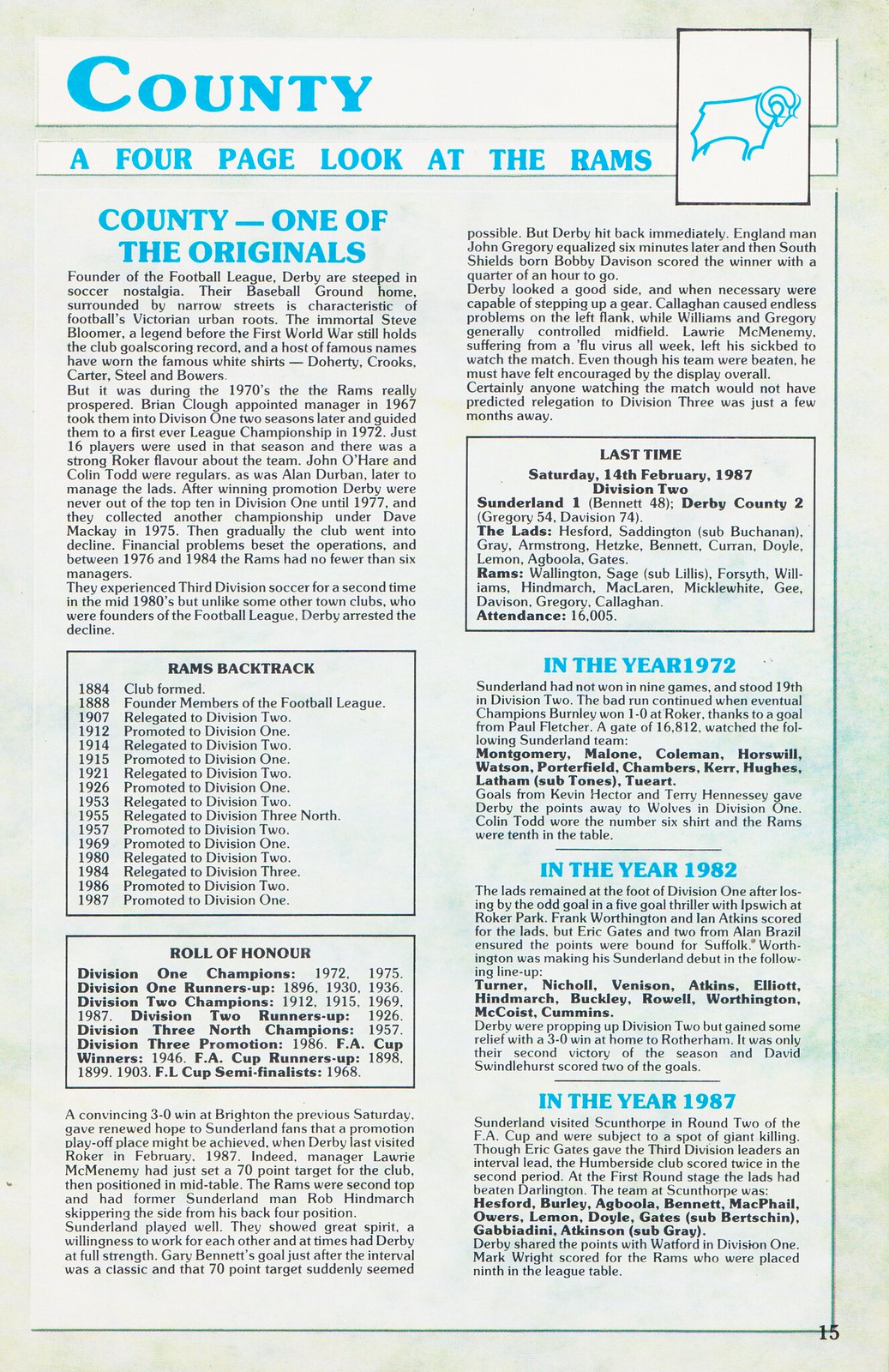The image showcases an old page from a multi-page document, possibly a magazine or newspaper, featuring the title "County: A Four-Page Look at the Rams." The page is approximately five by seven inches and marked as page 15 in the lower right-hand corner. Dominated by text, it includes aqua blue headings and small black lettering, largely unreadable in detail. The page is divided into two columns with several sections.

At the top, a drawing of a blue ram accompanies the title. The left column begins with the header "County: One of the Originals," alluding to the history of a football team named the Rams. Further down, a box titled "Rams Backtrack" displays various years and the team's league standings, hinting at its foundation in the 1800s and extending to 1987. Below is another box called "Roll of Honor," detailing significant divisional and championship achievements from the 1920s and 1930s.

The narrative continues into the second column, starting with a section called "Last Time," which focuses on the events of 1987. This is followed by smaller sections titled "In the Year 1972," "In the Year 1982," and "In the Year 1987," each highlighting notable occurrences and individuals from those years. The page appears to be part of a larger retrospective dedicated to the Rams within a historical context of county football.